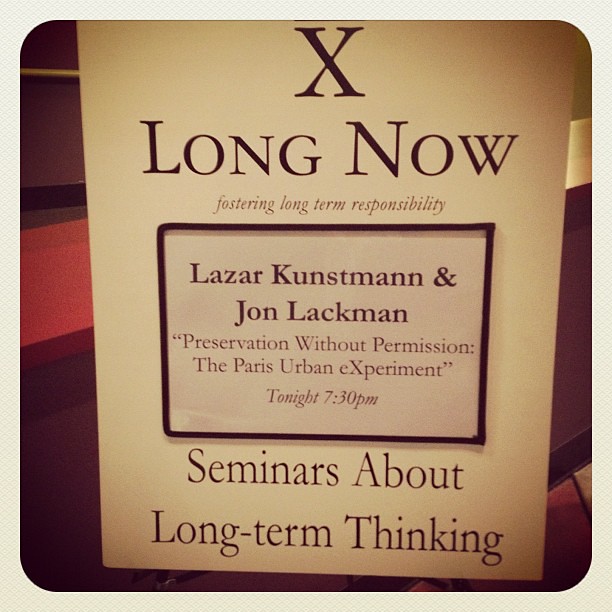This detailed photograph captures a notice stand situated in an indoor space, presenting a program encased in an off-white, textured digital frame with curved corners. The notice itself features a cream-colored card with a series of meticulously structured texts. Dominating the top is a large uppercase "X" in stark black, followed by the bold statement "long now," and underneath, in refined brown italics, the phrase "fostering long-term responsibility." Centrally placed within the notice is a bold black rectangle. Inside this, it prominently announces "Lazar Kunstman and John Lackmann," accompanied by the quoted text, "preservation without permission; the Paris Urban Experiment," specifying the event time as "tonight, 7.30 p.m." At the notice's foot, there is an additional caption in bold, "seminars about long-term thinking." The background reveals a red multicolored surface, contributing to an overall ambiance of depth and context. The photograph itself is tinged with a subtle brownish tint, enhancing the vintage feel of the depicted scene.